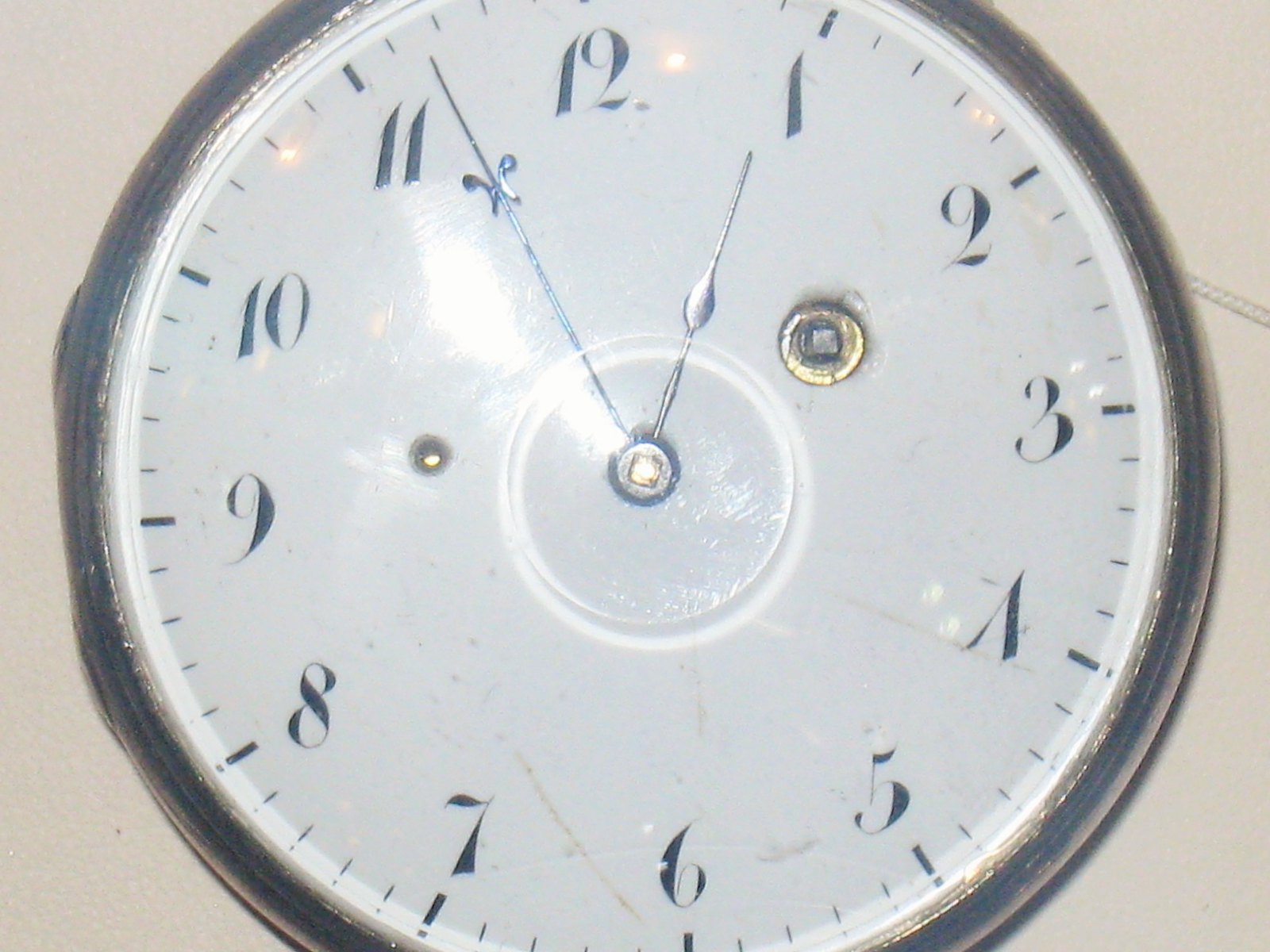The image is a first-person perspective, close-up shot of an older clock hanging on a wall. The circular clock has a worn and peeling silvery frame, indicating its age. The base of the clock is white with visible black numbers from 1 to 12 arranged in a clockwise manner, and thicker dash marks at each numeral position for clarity. The clock face is slightly reflective, suggesting it is covered by glass. At the center of the clock, a bolt holds the ornate hands: the hour hand is slender with a leaf-like design, and the longer minute hand features a small butterfly motif near its tip. The time displayed is approximately 12:56 or nearly 1:57, as the minute hand is just before the 57-minute mark, whereas the hour hand is positioned near the 1 but not quite there. The frame of the clock appears to be a tarnished metal, possibly black or bronze-brass, with slight reflective properties. The clock face also shows signs of aging, including faded areas and burn marks.